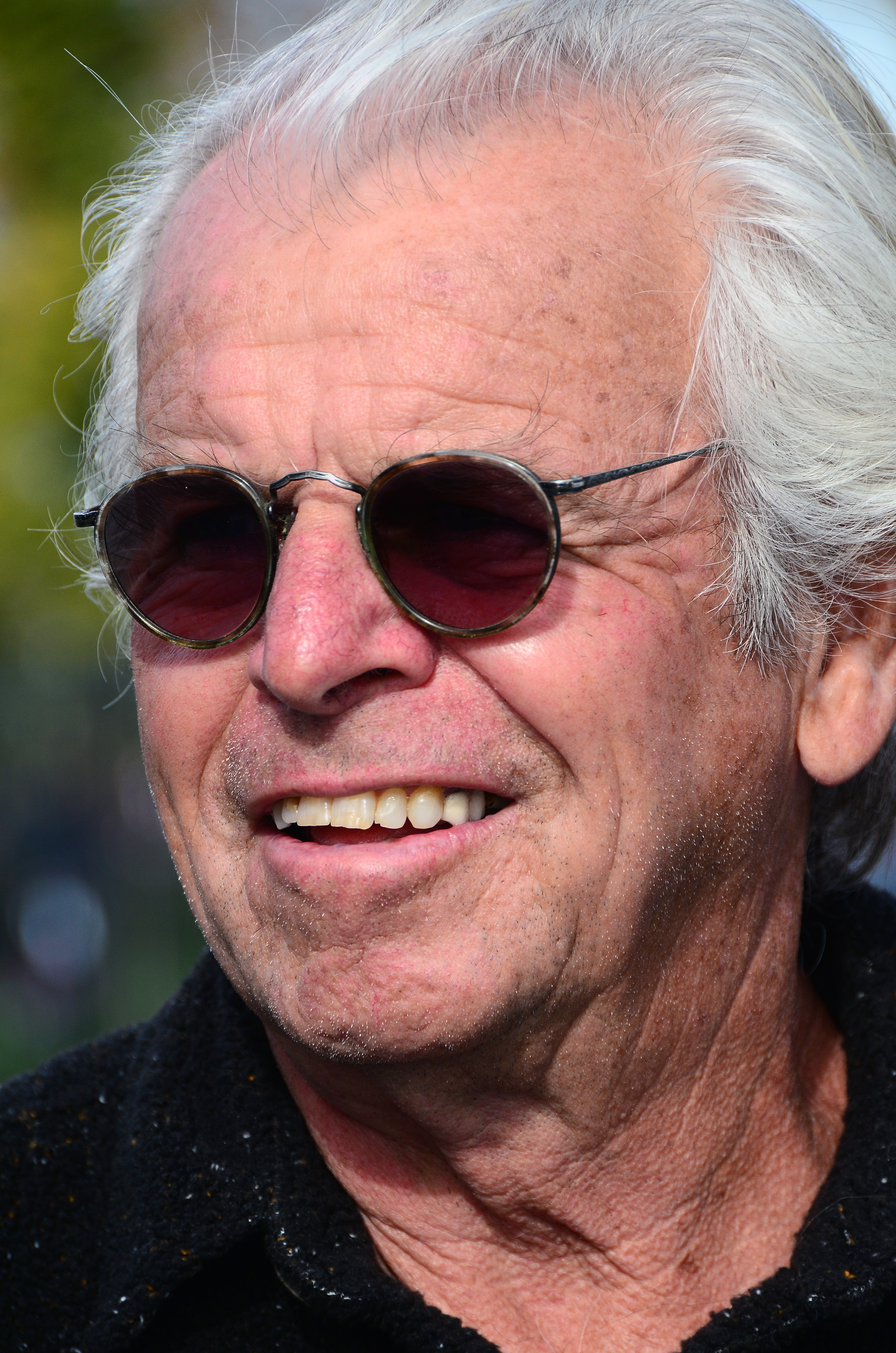The image features an older man with a familiar face, reminiscent of an old NFL football coach, though his identity is uncertain. His appearance is characterized by predominantly gray, slicked-back hair that is slightly balding on top, with occasional black strands visible. His hair is combed or blown back, and he has a little bit of stubble. The man's face is wrinkled and displays age spots, especially noticeable across his forehead and neck, which appears slightly droopy. He is smiling broadly, revealing his top row of teeth.

The man is wearing dark, round sunglasses and a black collared shirt adorned with small white and orange dots. The photograph is a close-up, focusing primarily on his face and neck, with the background appearing very blurry. Occasionally, hints of trees, gray, and blue can be discerned, adding a vague sense of the surroundings. His face is slightly angled, and he seems to be looking at something, enhancing the warmth of his smile.